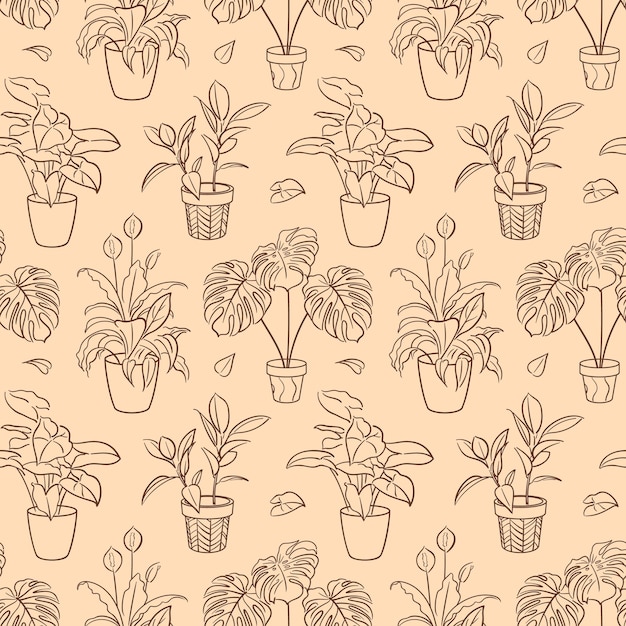The image depicts a beautifully simple yet elegant artist's sketch of various potted plants arranged in an array that resembles a potential wallpaper or tablecloth pattern. Set against a peach-colored background, the design features a series of monochromatic, dark gray or black outlines with no fill colors. The plants are organized in offset rows, creating a diagonal visual flow. They alternate between different types, including monstera, lilies, and others characterized by just stems and leaves. Each plant is depicted in a different style of pot—some plain white, others with swirly, diagonal, or geometric designs. Between most of the potted plants are heart-shaped leaves that fill the spaces, further contributing to the seamless, continuous feel of the pattern. Overall, the sketch art captures the essence of typical indoor house plants, with a mix of elaborate and simple pot designs, all set on a harmonious peach background.